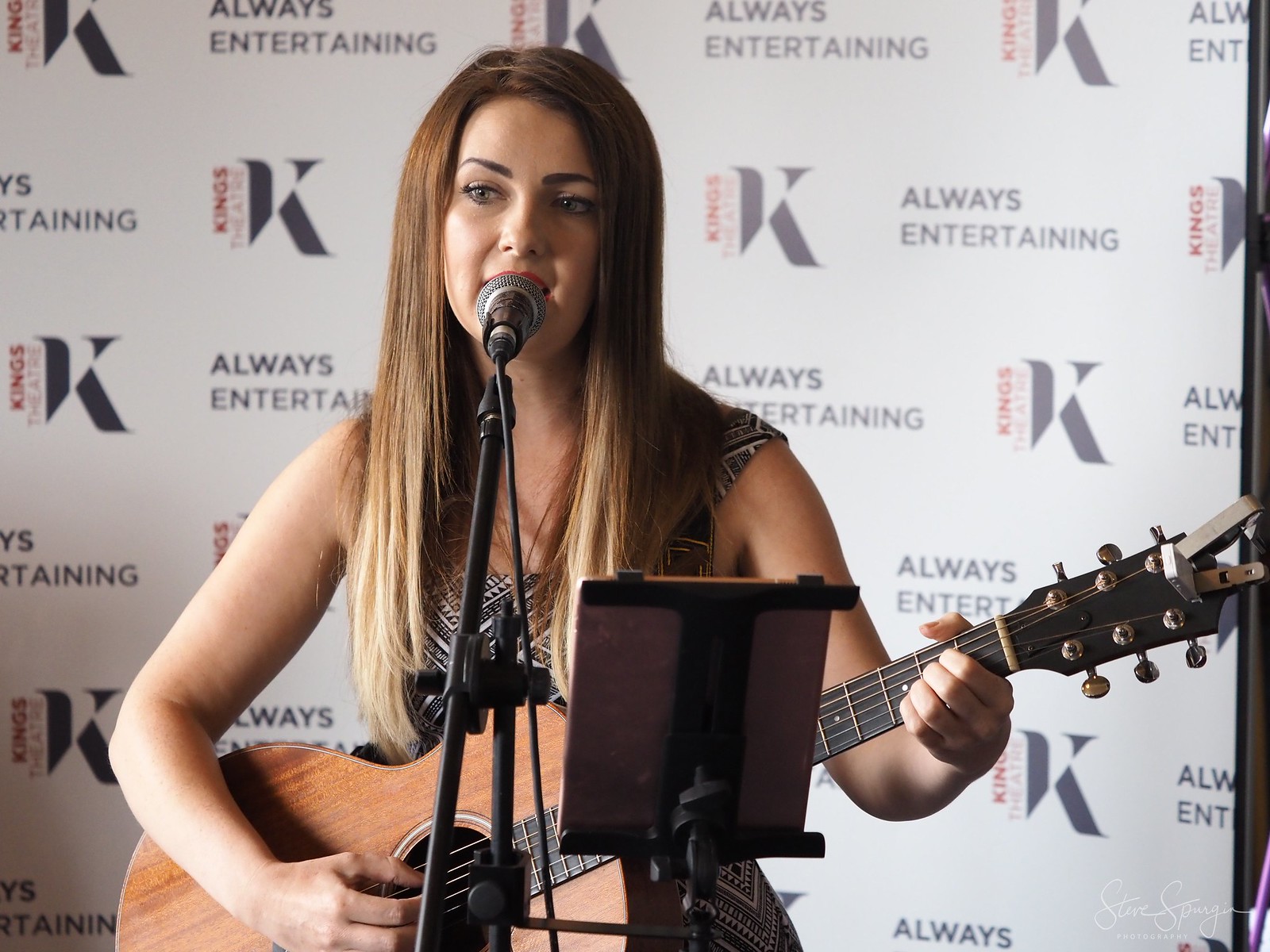In this scene, a young woman with long brown hair is performing a song. She stands in front of a microphone on a stand while holding and playing an acoustic wood grain guitar. She appears to be singing. A small stand in front of her holds a computer pad, likely displaying lyrics or sheet music. The stage backdrop is white with a graphic display featuring the words "Always Entertaining" and "Kings," along with a prominent large "K" logo. She is wearing a red and white dress and appears to have noticeable makeup. The setup suggests an unplugged acoustic set, adding a relaxed, intimate vibe to her performance.